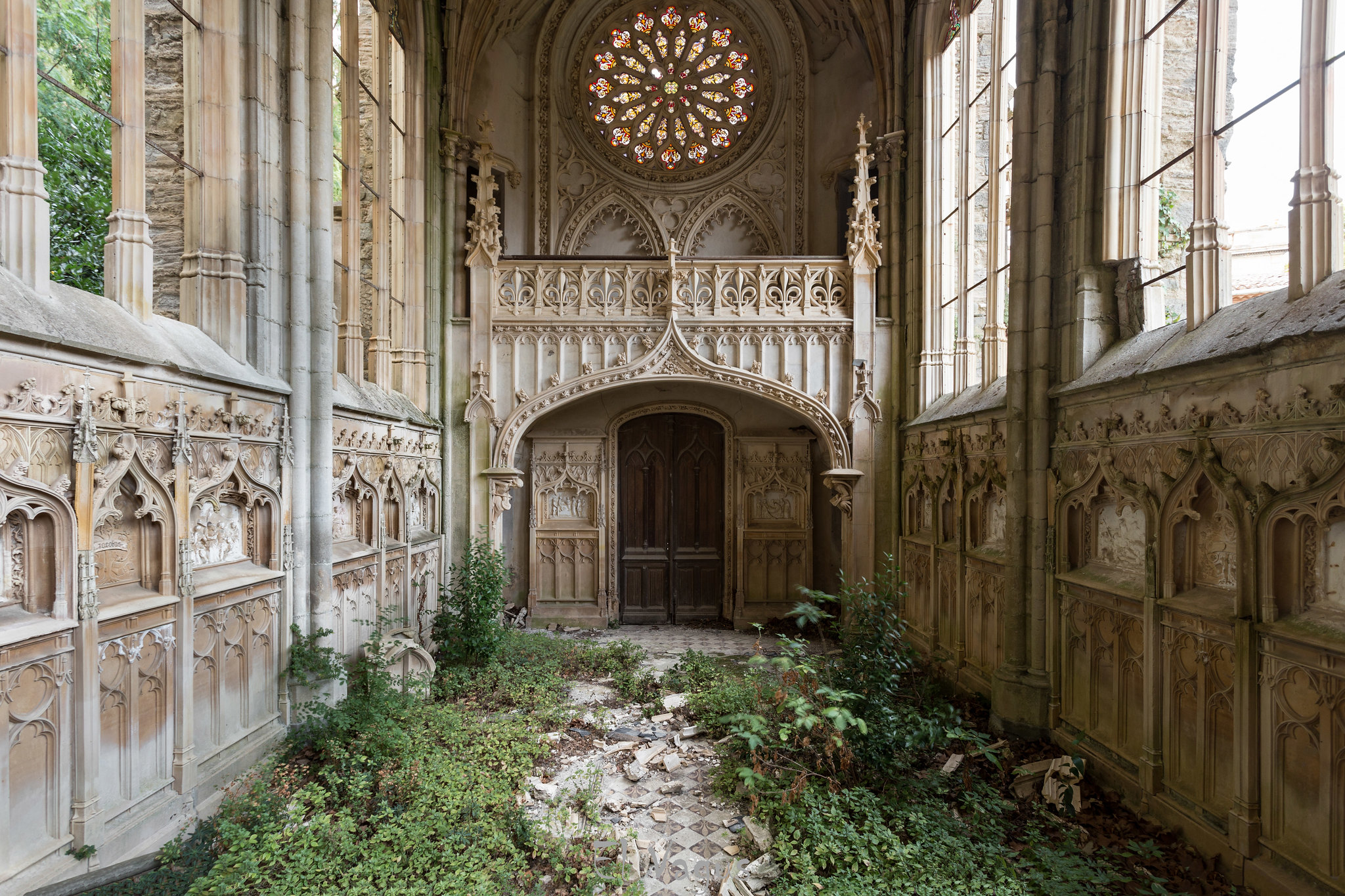This photograph captures the interior of a grand, historic church that has fallen into disuse. The foreground features an intricate, large brown door set within a prominent arched doorway, adorned with detailed stonework. Above the doorway, a stunning sun-shaped stained glass window gleams near the top of the frame, casting flickers of colored light into the dimly lit space. Just beneath the stained glass window, there's a narrow balcony that adds to the architectural grandeur.

Flanking the central view are towering stone walls lined with large windows, each surrounded by delicate carvings. These carvings create the illusion of tiny, puppet-show-like windows, adding a unique charm and texture to the structure. The floor, though mostly covered in patches of white and tan tiles, shows signs of neglect. Particularly along the left and right aisles, the tiles are broken, and the space is overrun with short green plants and bushes, indicating that nature is slowly reclaiming the area. Despite its state of disrepair, the church retains an air of faded elegance, hinting at its once-majestic past.